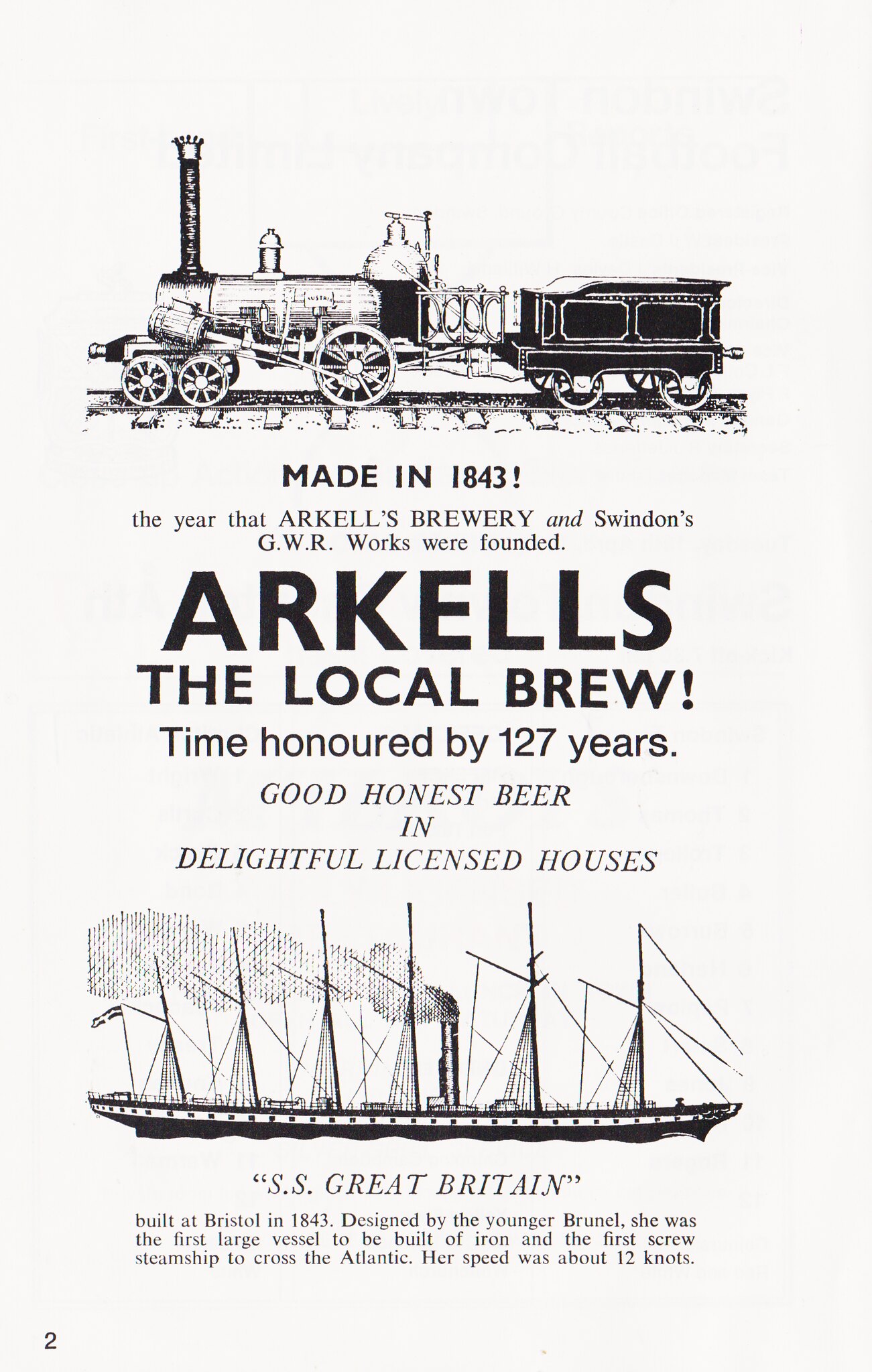This image is a detailed black-and-white vintage advertisement styled like a page from an old book, primarily promoting Arkell's Brewery. At the top, a locomotive engine pulling a train car is prominently displayed, emphasizing a historical period setting. Below the train, the text reads "Made in 1843," highlighting the founding year of both Arkell's Brewery and Swindon's G.W.R. works. The central portion features bold lettering stating "Arkell's," heralding it as the "local brew" with phrases like "Time honored for 127 years," and promoting it as "Good, honest beer in delightful, licensed houses." The bottom third of the image features a line art depiction of the SS Great Britain, the first large iron vessel and screw steamship to cross the Atlantic, designed by the younger Brunel and built at Bristol in 1843, with a descriptive paragraph detailing her historical significance. The overall imagery is rendered in shades of off-white, black, gray, and tan, with a central composition giving it a cohesive and classical aesthetic. The page is marked with the number two in the bottom left corner, adding to its vintage book-like appearance.